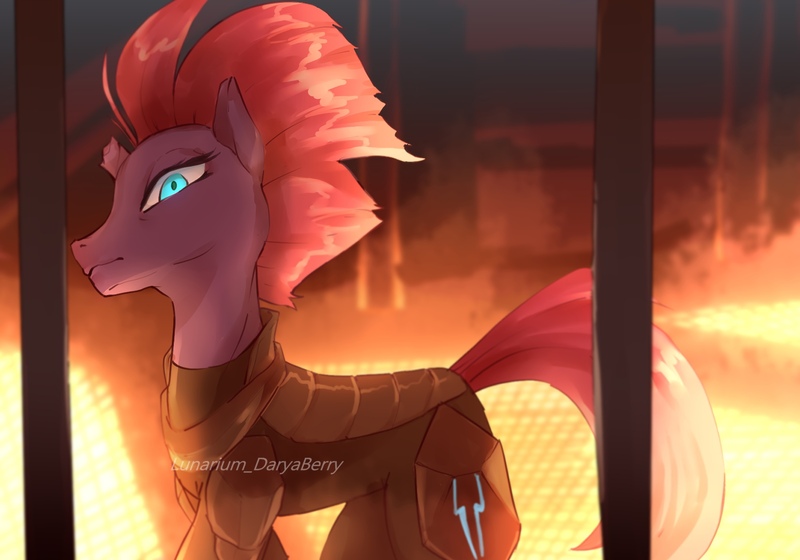This digital fan art appears to depict a My Little Pony-themed character, shown in a side view facing the left. The pony has a purplish-colored head with a large, almost glowing, light blue eye. Its red, spiked mane transitions into a wave towards the back, while its tail starts dark pink near the body and fades to a lighter shade towards the end, curling slightly to the left.

The pony is dressed in black armor covering most of its body, leaving the neck and head exposed, and features a brown saddle with a pouch on its back hip adorned with blue symbols. A hint of blue is visible on its back leg. The background is divided, with the lower portion displaying bright oranges and yellows suggestive of flames or lava, while the upper part is dark and industrial, resembling a factory or steel mill. Two vertical beams, one on the left and one in the middle of the tail, suggest a frame or industrial setting, adding depth to the environment. Overall, the scene exudes a slightly ominous and intense atmosphere.